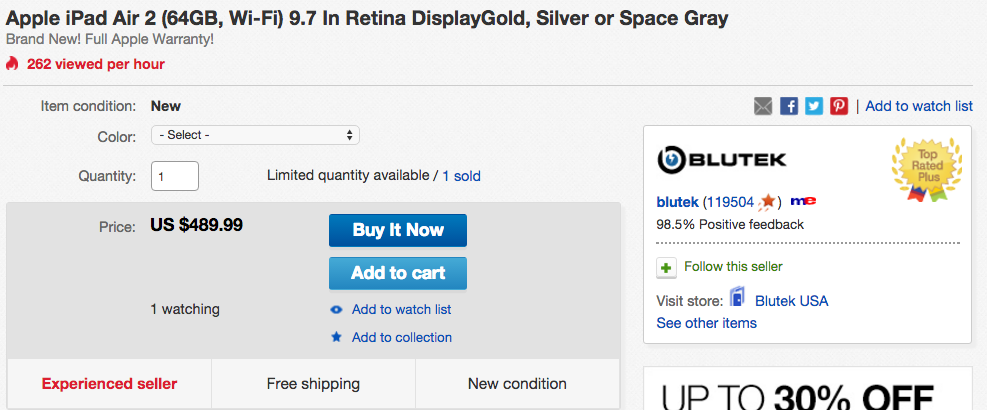The image is a product listing for an Apple iPad Air (4th Generation) with 64GB storage, Wi-Fi connectivity, and a 9.7-inch Retina display. The available color options are Gold, Silver, and Space Gray. The listing highlights that the product is brand new and comes with a full Apple warranty. Below the product description, it displays "262 views per hour" with a flame icon indicating its popularity.

A gray line separates this information from the details about the item's condition, which is "New." For the color selection, there is a dropdown menu where users can choose their preferred color. Below that, the listing mentions the quantity available, with the current selection set to one, indicating that there is limited stock with only one item sold so far.

The price of the iPad Air is $489.99, with two prominent action buttons: a blue "Buy It Now" button with white text, and another slightly different blue "Add to Cart" button with white text. The listing also notes that one user is currently watching the item and provides options to add the product to a watchlist or collection.

Additional details include the seller's information: a reputable seller with a 89.5% positive feedback rating (4 stars), and the username "blue_tek_119504". There are social media icons for sharing the listing on Mail, Facebook, Twitter, and Pinterest.